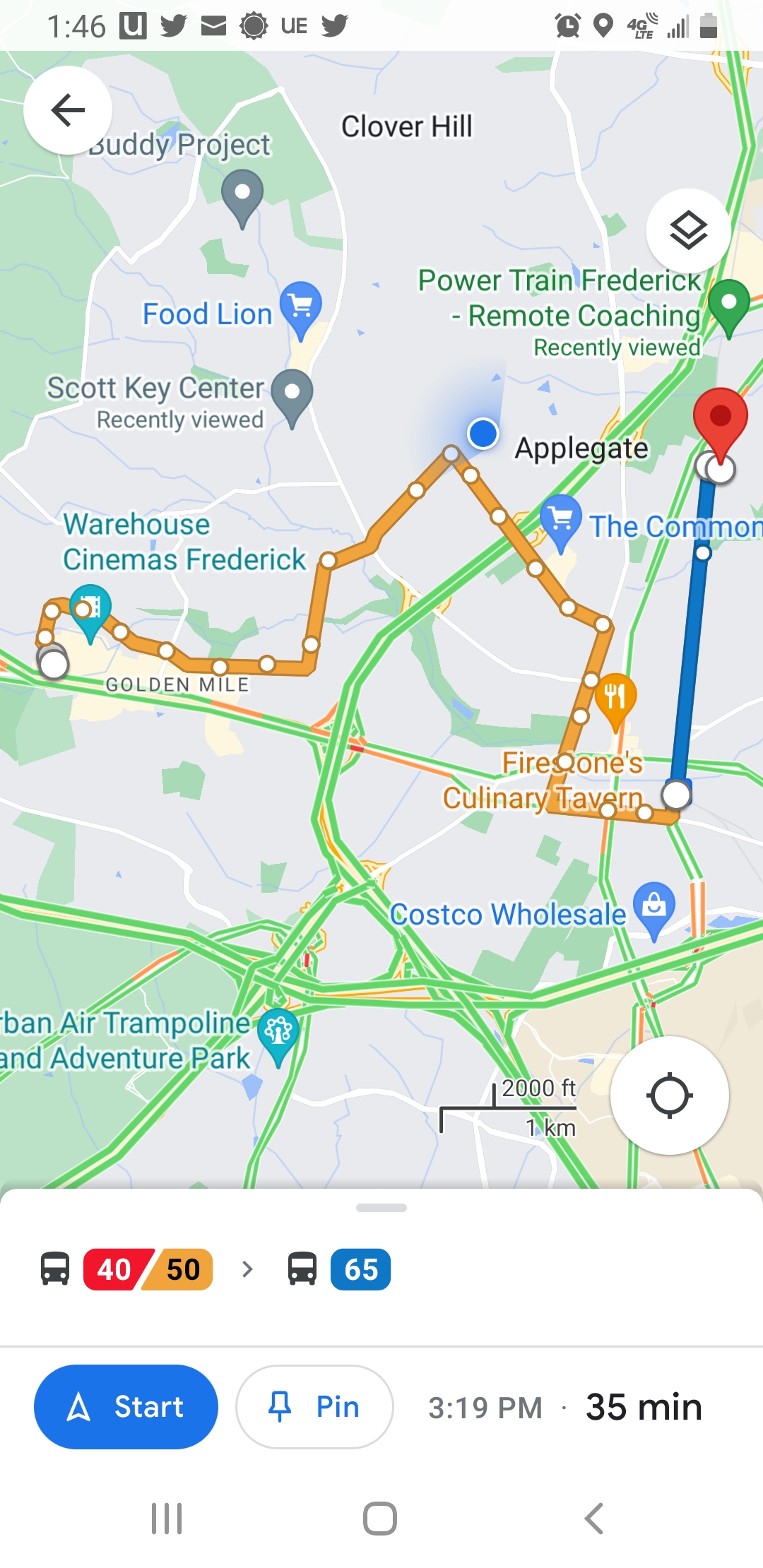The screenshot depicts a landscape-mode view of a navigation app on a phone. At the very top, a white banner displays various icons, including the Twitter and mail app icons, alongside indicators for battery level, cell signal strength, GPS location, the time (1:46), and a 4G LTE connection. The central portion of the screenshot shows a color-coded map, with green areas representing parks and streets, highlighted in orange for the designated route. This route appears to connect key locations such as Warehouse Cinemas Frederick and The Common. Additional business names and map pins are visible, indicating points of interest like Buddy Project, Clover Hill, Food Lion, Scott Key Center, Applegate, and Powertrain Frederick, among others. At the bottom of the screen, navigation options display estimated travel times by bus and car, showing durations from 40 to 65 minutes, a "Start" button, and a detailed time of arrival (3:19 PM) hinting at a 35-minute journey. The overall design blends practical navigation tools with relevant local information, enhancing the user's travel planning experience.